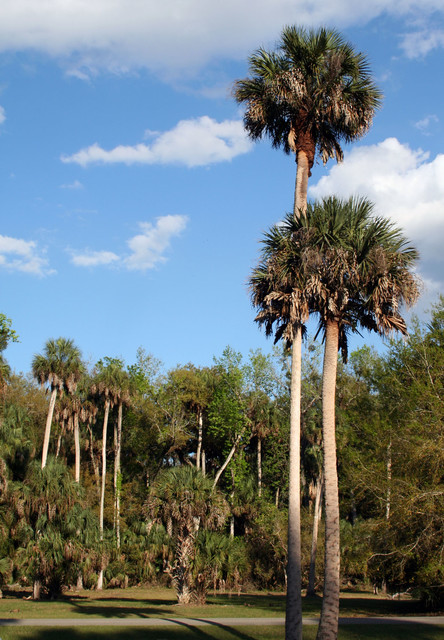This daytime image captures a serene, lush landscape reminiscent of a park or natural setting. The foreground features two prominent palm trees of varying heights; the tallest is on the left with a verdant, green crown accented by some brownish leaves underneath, while the slightly shorter one on the right mirrors this structure with its own slender trunk. This duo is set against a backdrop of numerous tall palm trees, creating a cohesive, green scene that stretches across the horizon. The sky, a pale blue canvas dotted with fluffy, scattered clouds, provides a tranquil setting for this vivid greenery. A concrete pathway begins at the bottom left and diagonally extends to the bottom right, bordered by patches of grass and dappled with the shadows cast by the overarching palms. The visual harmony of slim trunks, green crowns, and a clear sky suggests the photo was likely taken on a phone, capturing the vivid and refreshing ambiance of the area.